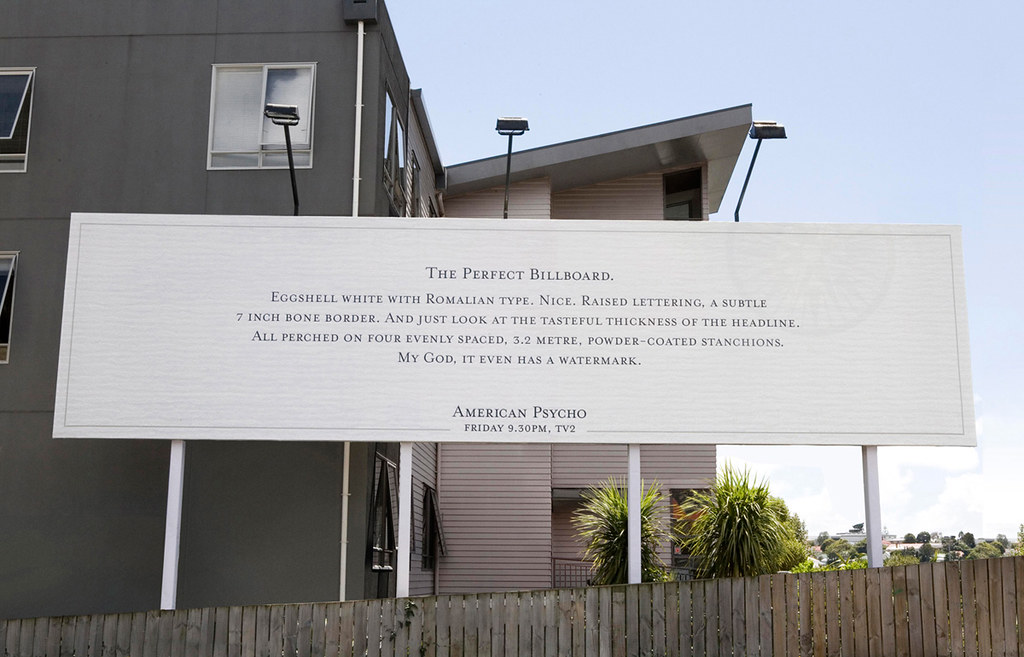This photograph, taken outdoors, shows a scene dominated by a cluster of buildings alongside a distinctive billboard. At the bottom of the image spans a long, beige-brown wooden fence with vertical slats, possibly aged and faded. Behind the fence, there's an olive greenhouse with three windows, two of which are partially visible, and a tan house that transitions from light gray to dark gray, and then to a mixture of light and dark browns. The second house features a slanted gray roof adorned with light green ferns and bushes, along with trees in the distance varying in shades of green. The background reveals a line of homes surrounded by more trees, with visible buildings in gray, brown, and white colors.

To the right side of the image, there's a large white billboard supported by four evenly spaced, 3.2-meter powder-coated stanchions and accented with three illuminating lamps. The text on the billboard reads: "The Perfect Billboard, eggshell white with Rommelian type, nice raised lettering, a subtle seven-inch bone border, and just look at the tasteful thickness of the headline." At the bottom of the billboard, it mentions, "American Psycho, Friday, 9.30 p.m., TV2," with a mention of a watermark adding a touch of authenticity. The sky above is a light blue, primarily overcast in the lower right corner, adding a calm backdrop to the setting.